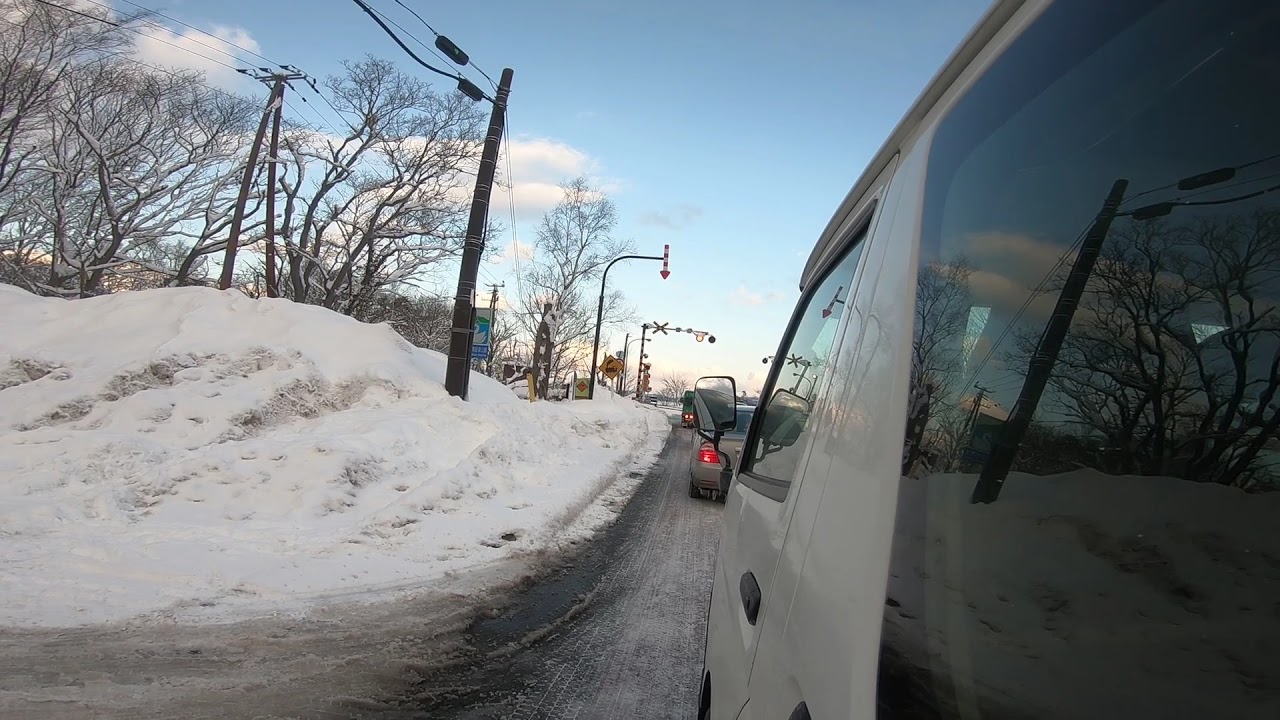This photograph captures a wintry scene featuring a white van driving on a snow-covered road. The image is taken from the driver's side of the van, providing a view of the driver's door and left side mirror. Ahead of the van is another vehicle, though its type is indistinct. The road is bordered by snow-laden ground, and beyond it, leafless trees are covered in a blanket of snow. Electrical poles, power lines, and traffic signals are visible on the left side of the road, with what appears to be a potential train signal further ahead. The sky above is a vibrant blue, dotted with white clouds, enhancing the cold, clear atmosphere of the day.